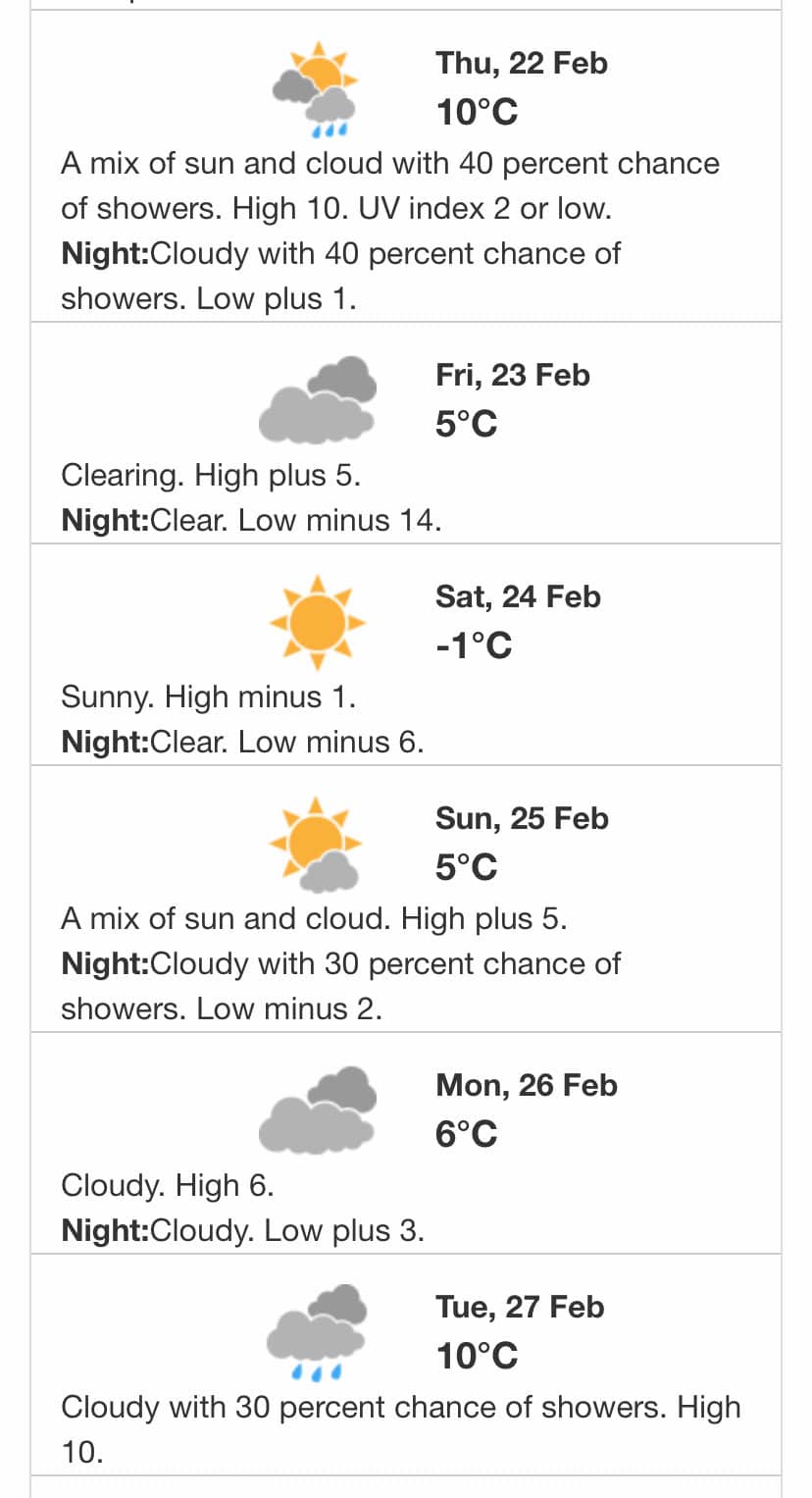The image presents a detailed weather report spanning several days, each displayed within its own white rectangle. 

- **Thursday, 22 Feb:** The icon features two clouds, a sun, and raindrops. The weather forecast predicts a mix of sun and clouds with a 40% chance of showers. The daytime high is expected to reach 10°C, with a UV index of 2 (considered low). At night, it will be cloudy with a continued 40% chance of showers and a low of 1°C.
  
- **Friday, 23 Feb:** The icon displays two clouds. The weather is forecasted to clear, with a daytime high of 5°C. The night will be clear with a low of -4°C.

- **Saturday, 24 Feb:** The icon shows a shining sun. The forecast is sunny with a high of -1°C during the day, and clear skies at night with a low of -6°C.

- **Sunday, 25 Feb:** The icon depicts a mix of sun and a cloud. The weather will consist of both sun and clouds, with a high of 5°C. At night, it will be cloudy with a 30% chance of showers and a low of -2°C.

- **Monday, 26 Feb:** The icon shows two clouds. The forecast is cloudy with a high of 6°C during the day and a low of 3°C at night.

- **Tuesday, 27 Feb:** The icon features two clouds with raindrops. The weather prediction is cloudy with a 30% chance of showers, with a daytime high of 10°C.